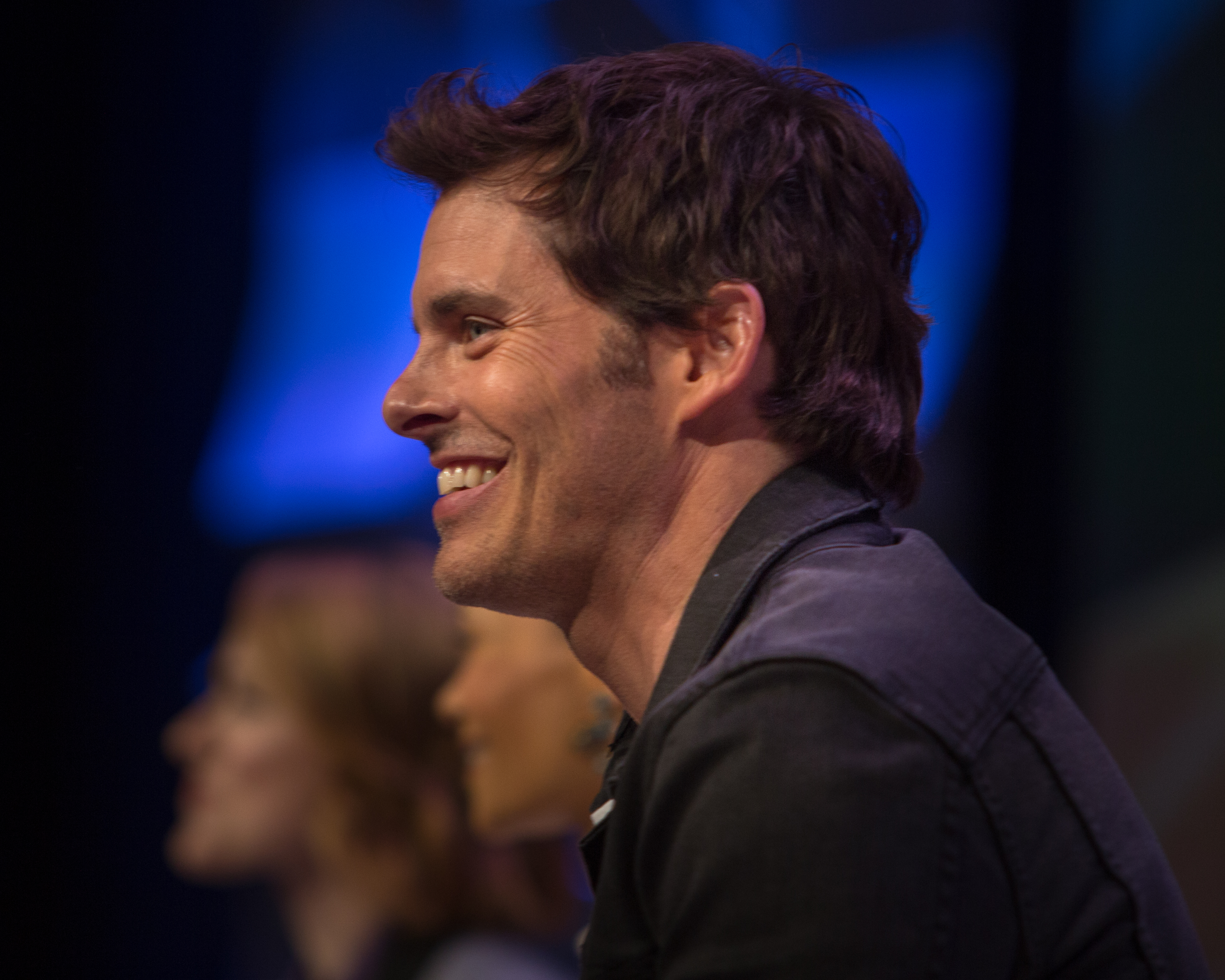In a close-up side profile, a man with a clean-shaven face and styled, fluffy brown hair gazes to the left. He wears a casual designer jacket in shades of black, navy blue, and possibly brown. He is smiling, revealing a sense of being impressed, with his blue eyes open and his left ear visible. The background is a blurred combination of dark blue and black, giving an indistinct but somewhat urban setting. There are also two blurred figures, likely women, in the background, further emphasizing the focus on the main subject. Overall, the photograph has no text, leaving the viewer to interpret the scene based on visual cues alone.